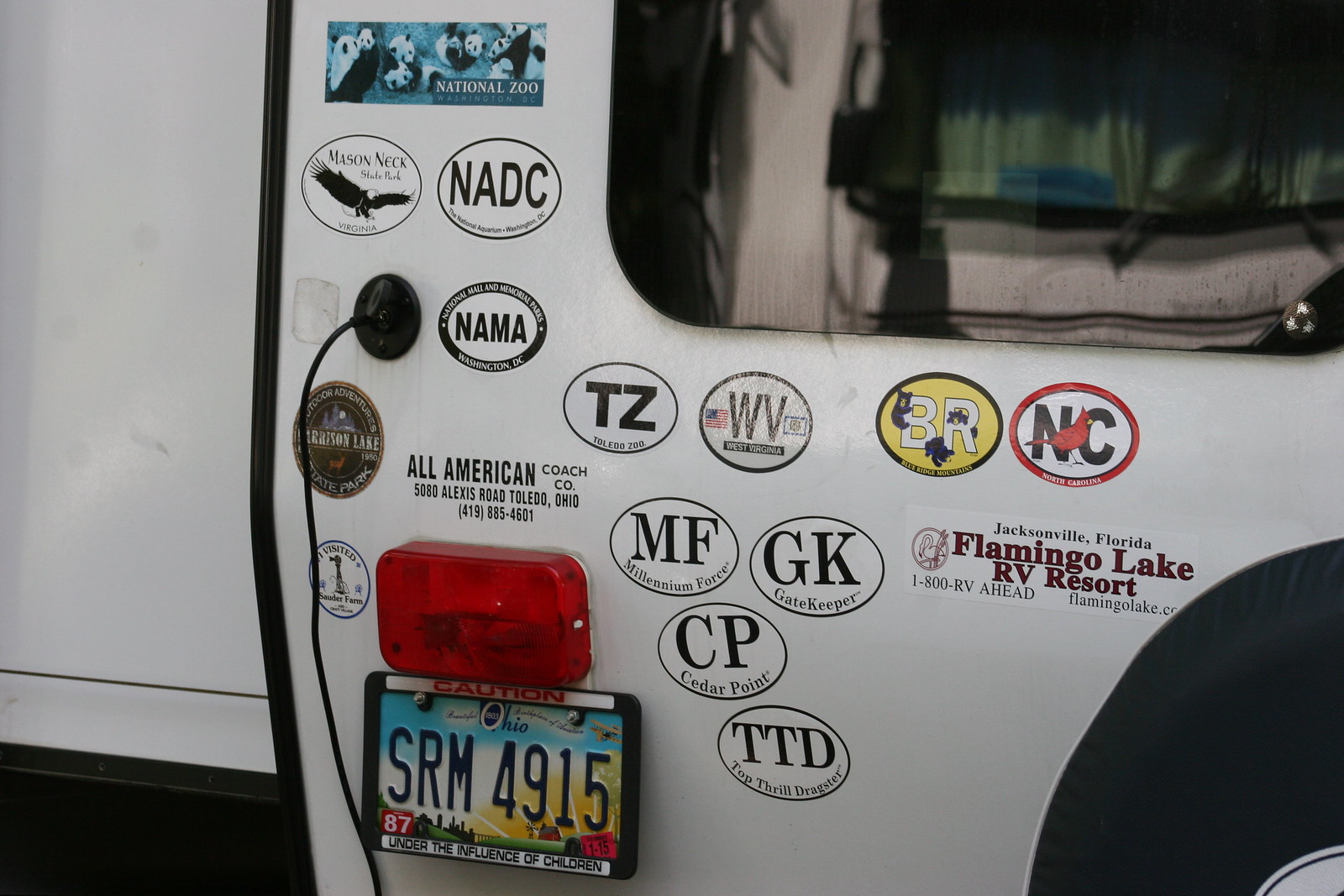This image depicts the side of a vehicle, likely a recreational vehicle or camper, plastered with a vibrant collection of 10 to 20 stickers showcasing various places and attractions visited. The white surface is adorned with black lines and numerous colorful stickers, each decorated with distinct pictures and text. Prominent among them, at the top, is a rectangular sticker featuring a panda and the words "National Zoo." Below it is a circular sticker with an eagle labeled "Mason Neck," and next to it, another circular sticker marked "NADC."

Additional circular stickers display abbreviations such as NAMA, TZ (Toledo Zoo), MF (Millennium Force), GK (Gatekeeper), CP (Cedar Point), TTD (Top Thrill Dragster), BR (Blue Ridge Mountains), and NC (North Carolina). Another notable sticker is a rectangular one inscribed with “Flamingo Lake RV Resort” and the information "1-800-RV-AHEAD, FlamingoLake.com," indicating its location in Jacksonville, Florida. 

At the bottom of the image is an Ohio license plate, SRM 4915, which bears the phrase "Under the Influence of Children" and the word "Caution" at the top. The license plate is colorful, suggesting the surface is indeed part of a vehicle. Also visible is a sticker from Outdoor Adventure State Park, Harrison Lake, partially obscured by a wire, and one from SAUDER Farm. The vehicle’s manufacturer, All-American Coach Company, provides additional details with an address in Toledo, Ohio, and a contact number: 419-885-4601.